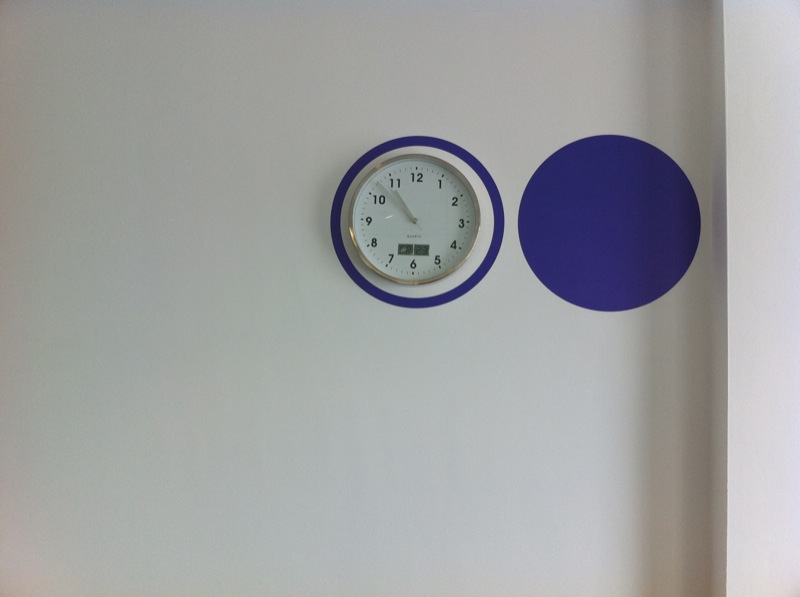The image features a white wall adorned with a clock. Positioned toward the middle of the right side of the wall, there is a dark blue circle. To the left of this dark blue circle, there is another circle outlined in dark blue, with a white interior. Within this white circle is a circular clock. The clock has a silver frame, a white face, and black numerals and hour markers. The clock reads 10:53, and all three hands—hour, minute, and second—are silver.